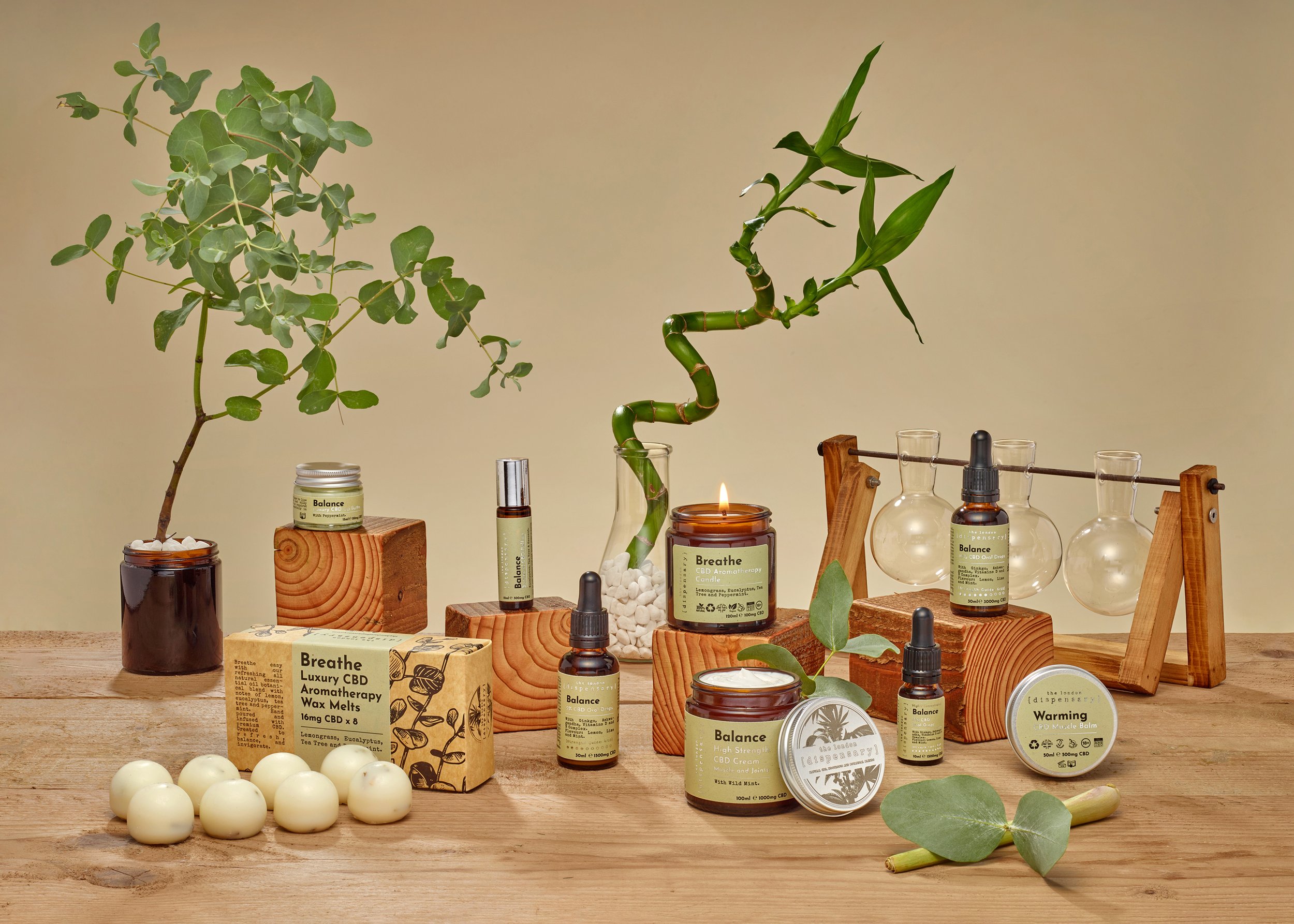This color photograph captures a meticulously arranged display of various natural and wellness products on a light-colored wooden surface, presumably a countertop or tabletop, with a light gray wall in the background. On the bottom left corner, there are two rows of four white, circular objects that are likely wax melts. Directly behind these, slightly to the right, is a rectangular package labeled "Breathe Luxury CBD Aromatherapy Wax Melts."

To the left and behind this package, there's a black pot with a sprawling plant featuring green leaves. To its right, a small wood block holds a tube of an unidentified product. Another wood block, positioned further back, supports a bottle with a dropper lid. In front of these, closer to the viewer and slightly to the right, is a glass jar with a thick green stem that curves elegantly, flanked by a candle in a jar—one lit and one unlit with its lid placed beside it. Additional wooden blocks house other products, including candles labeled "Breathe," "Balance," and "Warming."

A wooden rack with vertical side pieces and a horizontal connecting bar at the top is situated at the back right, holding three glass containers with tube-like tops. In front of this stand, there's a small canister and two green leaves, partially obscuring a small yellowish cylindrical item behind them.

Overall, the display exudes a calm, natural aesthetic with colors primarily revolving around green, brown, beige, and other earthy tones, accentuated by bamboo leaves scattered across the scene.